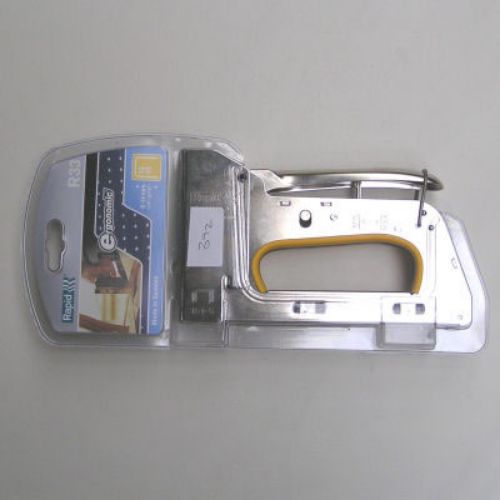The image features a staple gun positioned centrally and lying sideways against a dark gray background. The staple gun, still in its packaging, is designed to be handheld and is roughly rectangular in shape. The tool itself is predominantly silver metallic with a black or dark silver body and an orange accent around the handle area. The packaging features a plastic front with a cardboard backing. On the left side of the package, the label reads "Rapid R33" in white text. The packaging also includes a photograph of the staple gun in use, over a floor surface, with segments highlighted in blue and additional orange logos. The colors visible in the image include gray, silver, yellow, blue, green, white, black, and a bit of orange. The overall setting and style suggest a home improvement context, reminiscent of displays in stores like Home Depot or similar retail environments.